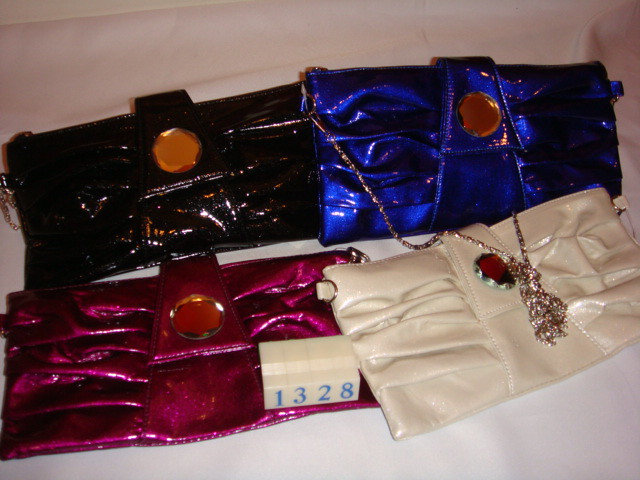On a soft, light pink cloth display, four elegant ladies' handbags are showcased, each sharing the same sophisticated shape and style but differing in vibrant colors. These handbags, suitable for dressy occasions, feature an amber-like, circular gold plate in the center of each flap. The colors stand out distinctly: a shimmering hot pink, a stunning dark sapphire blue with an accompanying shiny, chrome-like silver strap, a pristine white, and a very dark brown, almost black bag that exhibits a high gloss. Additionally, there is a small white tag in front with the numbers "1328" inscribed in blue, enhancing the meticulous arrangement.